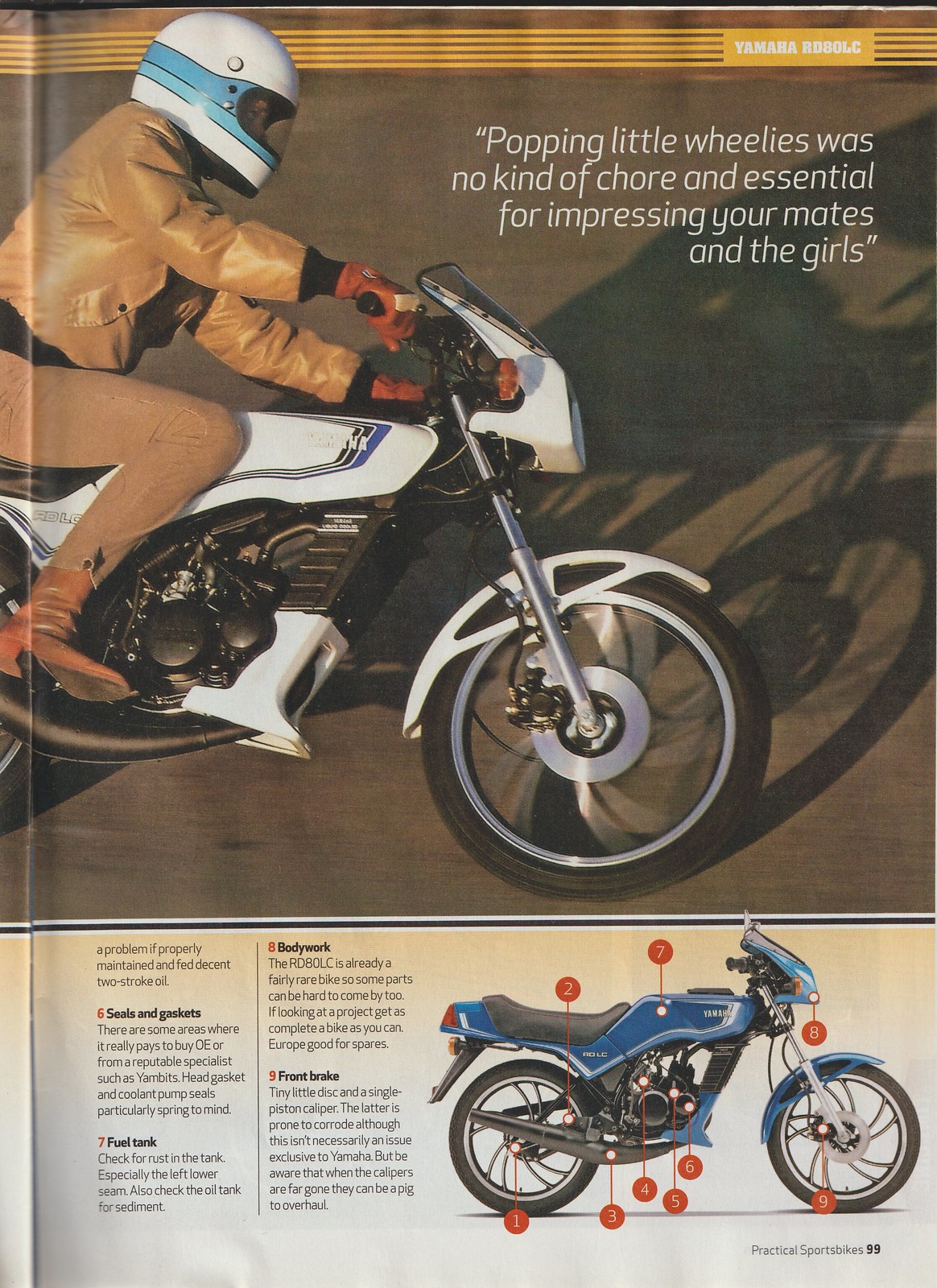The image is a magazine page advertising a white motorcycle, prominently featuring a photograph that occupies the top two-thirds of the layout. In this photograph, a rider can be seen in motion, riding on a black-top road. The rider is stylishly dressed in tan-colored leather boots, tight-fitting brown denim pants, and a brown leather jacket with front pockets near the stomach. They are also wearing darker brown leather gloves gripping the black handles of the motorcycle, and their head is protected by a white helmet with blue stripes that match the bike. Overlaid on this dynamic image is a white text that reads, "Popping little wheelies was no kind of chore and essential for impressing your mates and the girls."

Below the photograph, the bottom one-third of the page features various informational details about the motorcycle. There’s a border at the top of this section in yellow with the text "Yamaha Roadblock." The white background beneath contains text headers such as "Seals and Gaskets," "Fuel Tank," "Bodywork," and "Front Brake" in black, pointing to different parts of a diagram of a blue bike. Also visible on the left side of the page is the seam where the middle of the magazine is located.